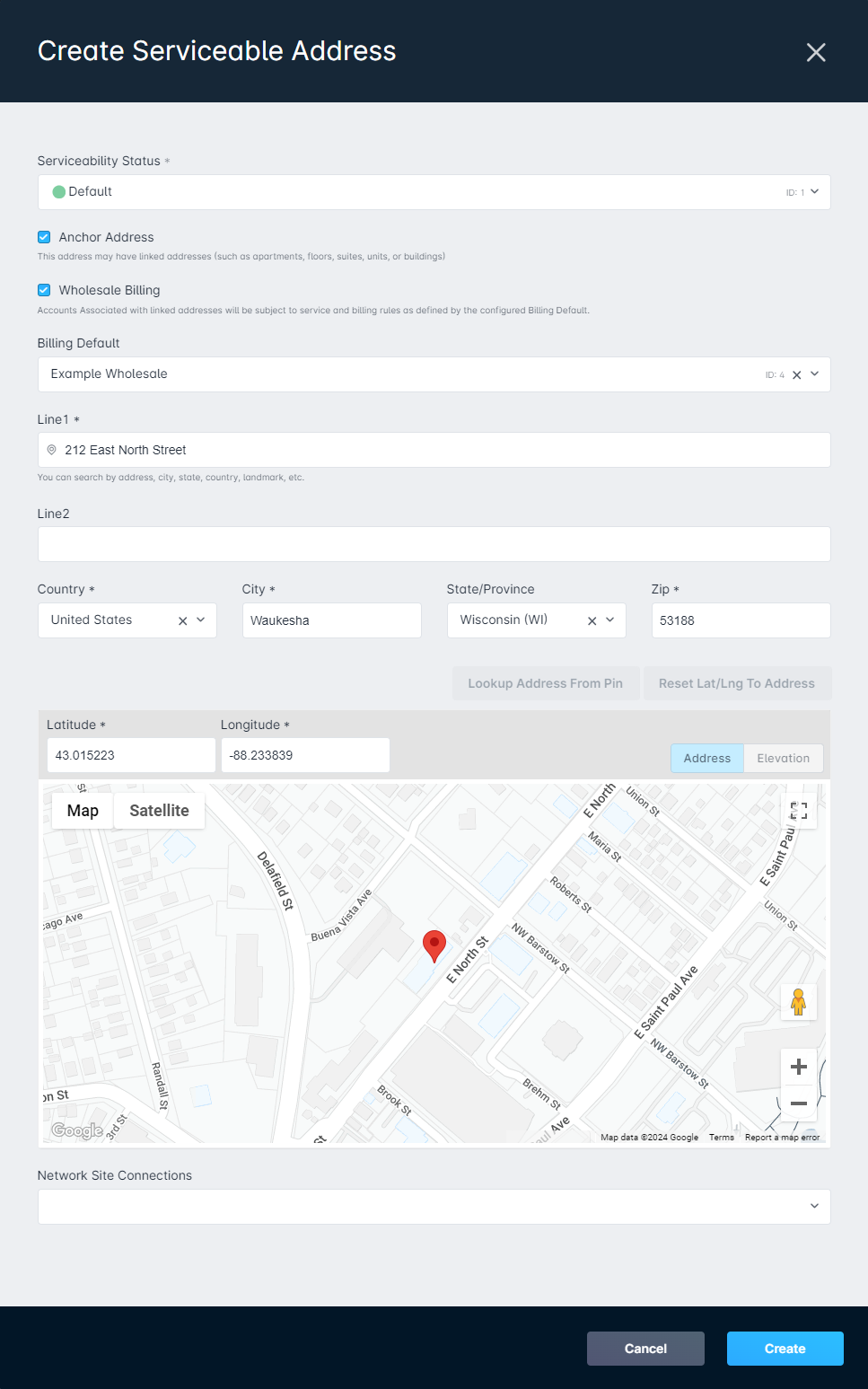**Detailed Caption:**

The image displays a user interface with a header titled "Create Serviceable Address," which is presented in white text on a black and navy blue background. Below the header, there are multiple drop-down boxes for different input fields. 

- The first drop-down is labeled "Serviceability Status," which is displayed in a white box with a green dot indicating 'Default' status.
- Directly beneath this, there are sections for "Anchor Address" and "Wholesale Billing," each accompanied by a brief description. The "Anchor Address" section is currently marked with a blue checkmark and includes the note: "This address may have linked addresses such as apartments, floors, suites, etc." 
- The "Wholesale Billing" section describes that accounts associated with the linked address will be subject to services and billing rules as defined by the configured billing date. Currently, it shows a placeholder example for "Wholesale".

Further down, the interface provides fields for entering specific address details:
- Line 1 shows an address: "212 East North Street."
- Line 2 is left blank.
- The "Country" field features a drop-down menu, currently selected as "United States."
- Adjacent to the country, "Waukesha" is listed under the city/town input.
- The "State/Province" field shows "Wisconsin," and the Zip Code is "53188."

Additionally, the interface includes geographical coordinates displayed as latitude and longitude numbers, alongside a map with a pin placed north of East North Street. The map functionality allows toggling between "Map" and "Satellite" views via a top-left corner button, and zooming in or out using plus (+) and minus (-) buttons.

At the bottom right of the interface, there is a blue "Create" button, while to the left of it, there is a gray "Cancel" button.